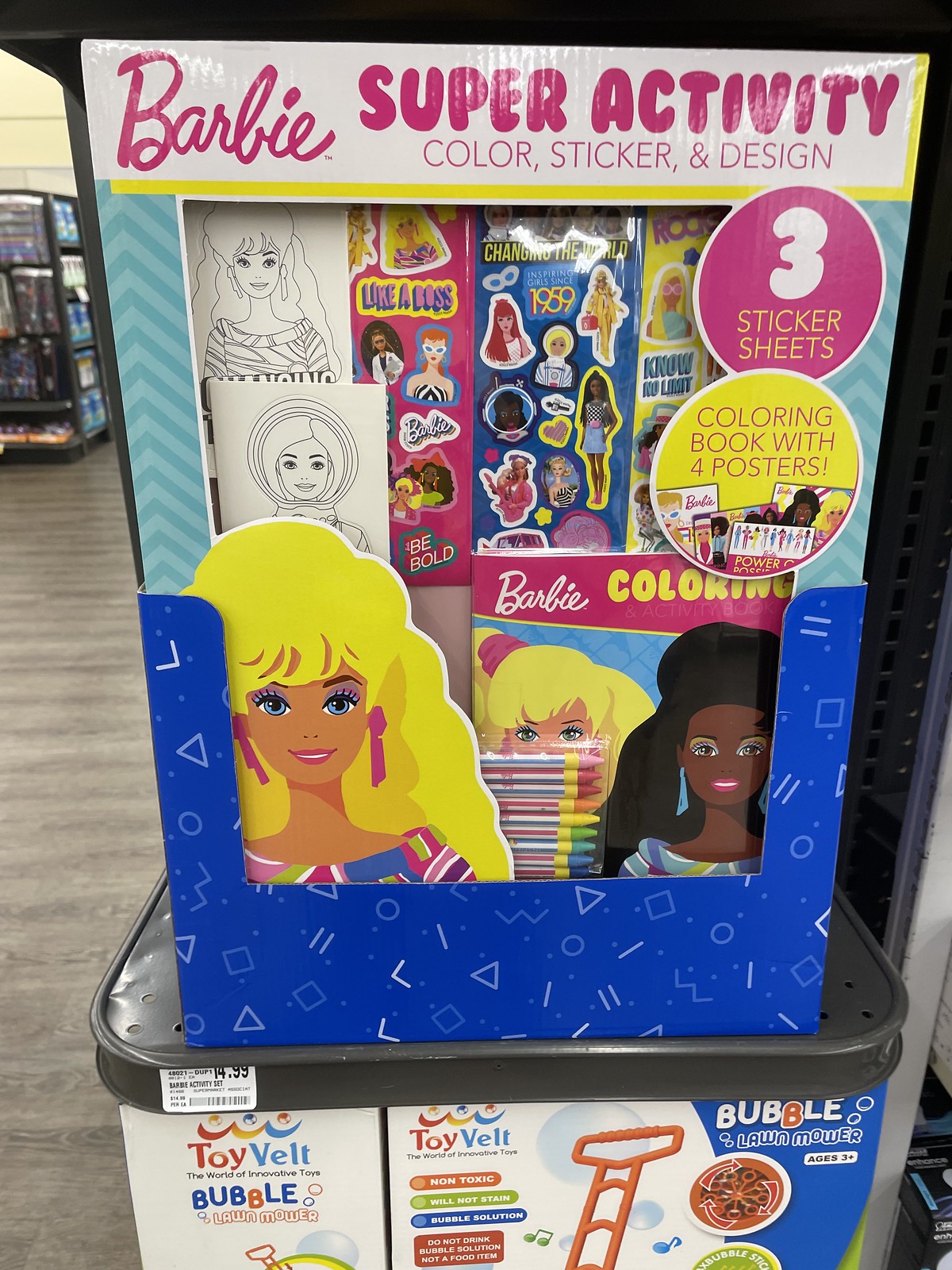The image depicts a vibrant retail kiosk within a store, dedicated to Barbie Super Activity Color Sticker Design. The kiosk features a prominent glass panel edged with a blue border and topped with white and pink text proclaiming "Barbie Super Activity Color Sticker Design." In the top right is a pink circle that declares "Three Sticker Sheets," and below it, a yellow circle announces "Coloring Book with Four Posters." Inside the glass, various Barbie-themed activity kits are displayed, including sticker sheets, coloring books, crayons, and other creative materials. The display includes an illustration of Barbie on the bottom left, dressed in multicolored clothes with earrings, alongside a cover image of an African-American Barbie. The kiosk sits atop what seems to be an ice cream chest, surrounded by other toys, including a partially visible bubble-blowing lawnmower designed for young children.